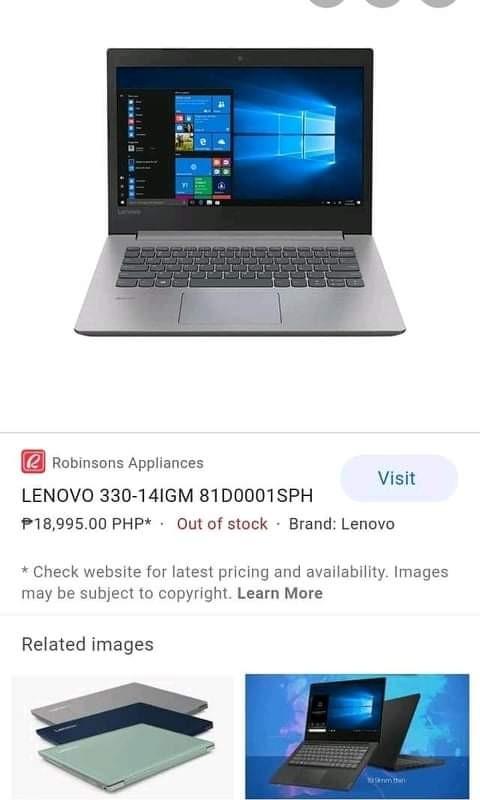At the top of the image, there is a photograph of an open laptop with its screen facing the viewer. The laptop's wallpaper features an open window allowing light to pour in from the left side. The screen also displays a menu and a few pop-up windows on the left side. The laptop itself has a steel-colored gray surface with a black keyboard. Below this image, there is a detailed product description: "Robinson's Appliances, Visit, Lenovo 330-14IGM, 81D0001SPH, 18,995 PHP, out of stock, brand Lenovo, check website for latest pricing and availability, images may be subject to copyright, learn more, related images."

Under this, on the left side, there is a photo of three closed laptops stacked atop one another. The top laptop is dark gray, the middle one is black, and the bottom one is sage green. To the right, there is another image displaying two open laptops. The laptop on the left is facing the viewer, while the one on the right shows the back part of the device. The background of the entire image is blue, with some indistinct white text that is too small and blurry to read clearly.